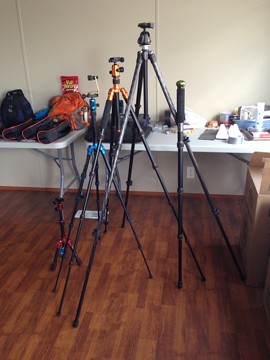The image depicts a room with a wooden floor and a white-paneled wall accented with brown trim at the bottom. On the floor, various tripods of different sizes are closely grouped together. The tallest tripod is black and centrally located, standing prominently above the others. To its left, there's a slightly shorter tripod with a golden-orange top and black legs, followed by another shorter tripod with a bright blue metal top and black legs. Further to the left is a tiny tabletop tripod featuring red and black details. In the background, two white folding tables are positioned against the wall, holding various pieces of equipment, some of which are out of focus. On the left table, there are black cases with red linings and gray and orange bags. To the right of the tripods is a tall cardboard box with open flaps. Additionally, the room contains a white heating vent on the floor and some scattered items, including stacks of paper and white boxes, adding to the busy atmosphere.